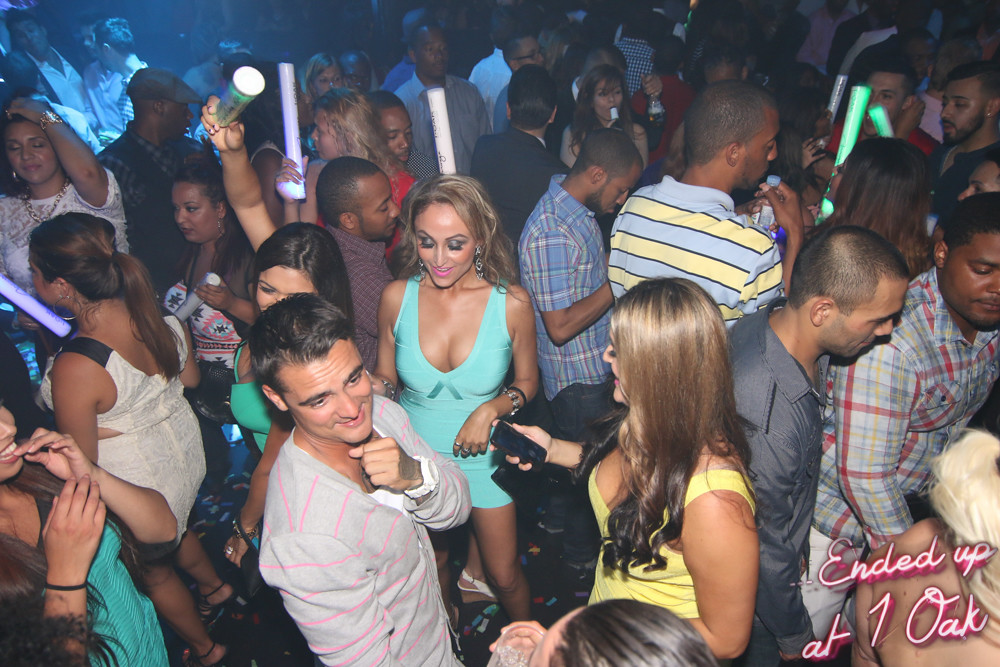The photograph captures a lively club atmosphere at One Oak, highlighting a room filled with dozens of young people, primarily in their 20s and 30s. The overall setting is dark, accentuated by sparse, club-like lighting that enhances the mood. The women are dressed in stylish dresses, often with makeup, while the men are seen in nice, casual shirts. Many attendees are holding up large, glowing sticks, contributing to the festive ambiance. In the background, a few individuals can be seen enjoying drinks, possibly beer. The image is marked by white neon text in the bottom right corner that reads "ended up at One Oak", solidifying the venue's identity.